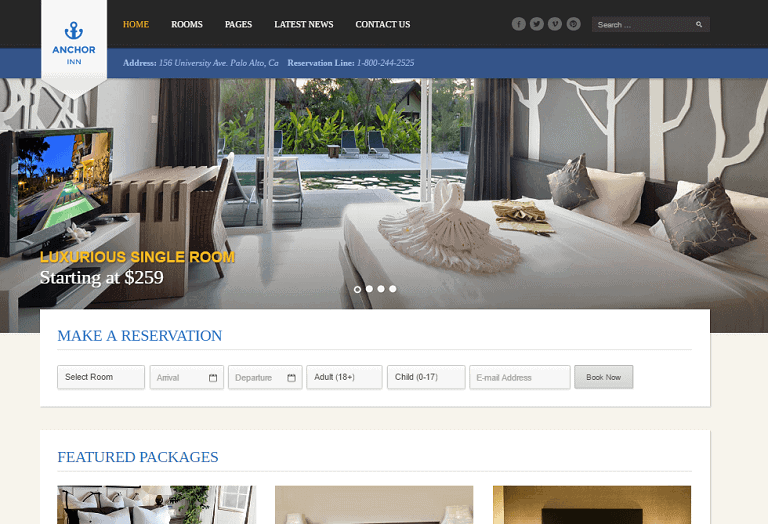Website Overview of Anchor Inn:

The webpage for Anchor Inn is presented with a sophisticated layout, showcasing a photograph of a luxurious single room. Beyond the room, an inviting pool area with lounge chairs, lush trees, and nearby buildings creates a serene backdrop.

At the top of the page, a sleek black navigation bar includes the following options: "Home," "Rooms," "Pages," "Latest News," and "Contact Us." On the right side of this bar, social media icons for Facebook and Twitter, along with a share button and an unidentified icon, are displayed. A search bar also features on this black band.

Beneath the black navigation bar, a blue strip provides key information: "Address: 156 University Avenue, Palo Alto, California." It also lists the reservation line number: "1-800-244-2525."

Prominently displayed, a downward-pointing tab labeled "Anchor Inn" extends past the blue strip. This tab features an anchor icon and the text "Anchor Inn," both in blue.

Overlaying the room photograph, a caption reads: "Luxurious single room starting at $259," emphasizing the room's high-end appeal.

Below the photograph, a white rectangular section offers a user-friendly reservation interface. It includes fields for selecting "Room," "Arrival," and "Departure" dates (each equipped with a calendar), specifying the number of adults (18+) and children (0-18), entering an email address, and finalizing the booking with a prominent "Book Now" gray button.